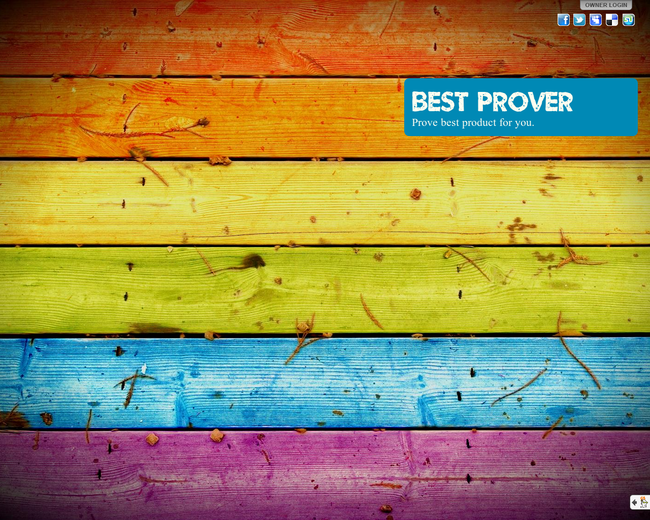The image is a photorealistic depiction of a series of six horizontally stacked planks of wood, each stained a different color of the rainbow, sequentially from top to bottom: red, orange, yellow, green, blue, and purple. Each plank is of the same size but exhibits slight pockmarks, different textures, and a variety of small holes and staples, with dirt, grass, and pine needles scattered over them. In the upper right corner, there is a blue rectangle with white text reading "Best Prover," followed by smaller white text that reads "Prove Best Product For You." Above this blue box is a button labeled "Owner Login," and a row of five icons representing major and smaller social media platforms, starting with Facebook and Twitter on the left. The details suggest it might be an element of a web design template, possibly indicating login options and social media links for user interaction.